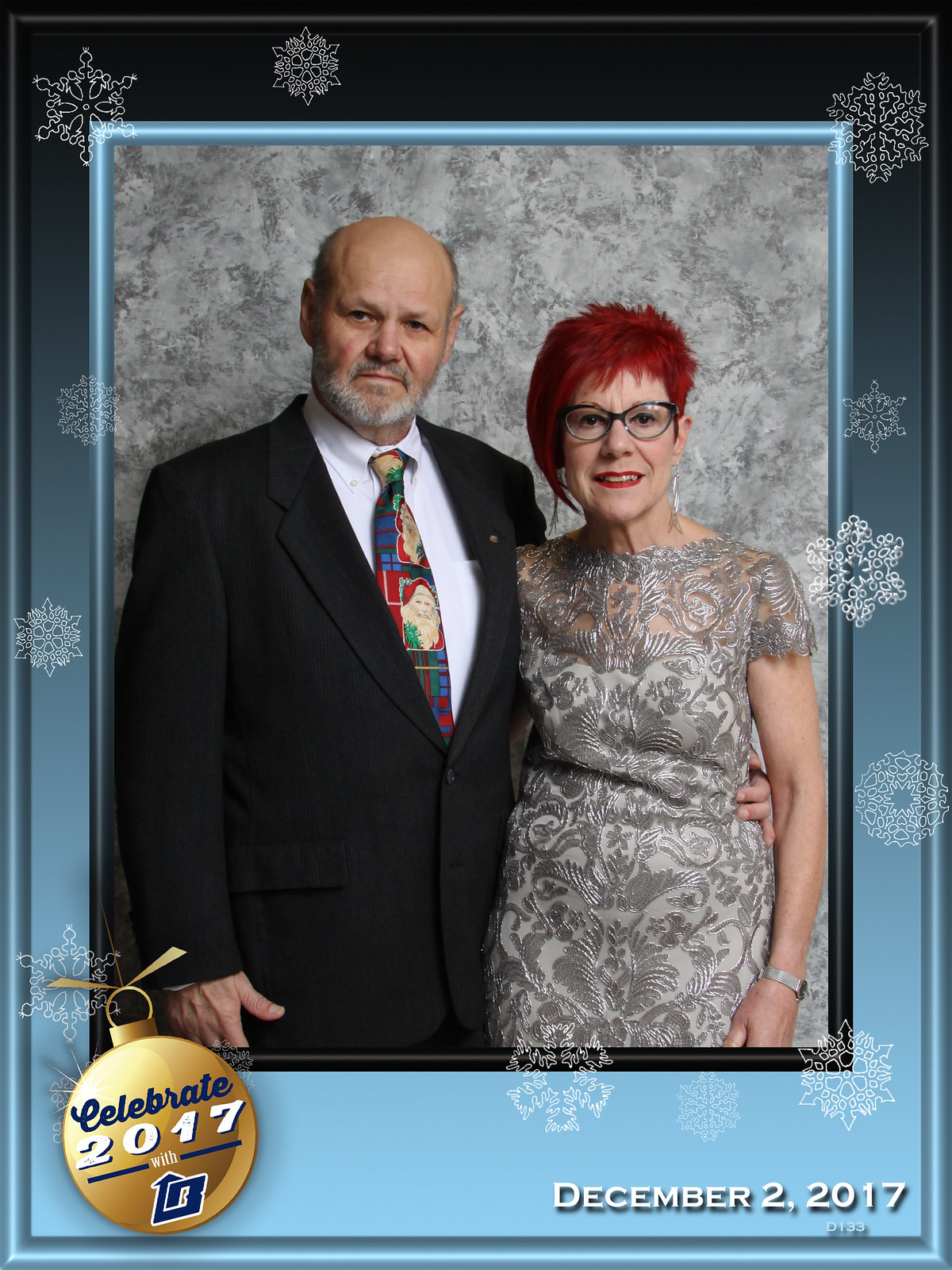This is a detailed portrait of an older couple, possibly taken for a Christmas card or anniversary celebration in 2017. The man, standing on the left, is dressed in a black suit with a white button-down shirt and a festive Christmas tie featuring Santa Claus and other colorful designs. He is bald, with hair on the sides, and has a white beard. He stands with his arm around the waist of the woman beside him. She wears glasses with black rims and has striking, short, spiky red hair styled to one side. Her attire is a elegant silvery beige lacy dress with a floral pattern. The background of the photograph is a splotchy gray, and the picture is framed with a shiny blue frame that fades from dark at the top to light at the bottom, adorned with snowflakes. A golden ornament in the corner bears the words "Celebrate 2017" in blue and white letters. Additionally, the date "December 2, 2017" is inscribed at the bottom of the frame.